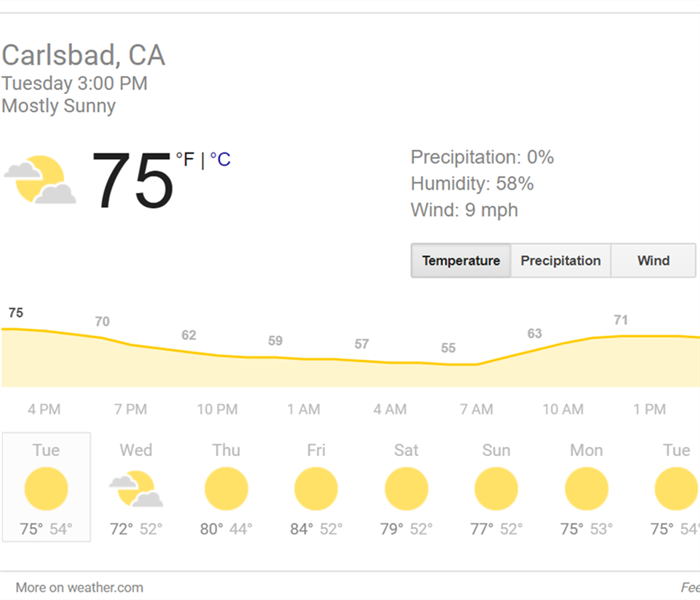A screenshot of a weather forecast from weather.com is presented against a white background. Two thin horizontal gray lines frame the top and bottom of the forecast information. Below the top border, the location "Carlsbad, CA" is displayed in a grayish font, alongside the current time "Tuesday 3pm" and the weather condition "Mostly Sunny."

The forecast prominently features a yellow sun icon partially obscured by clouds at the top left and bottom right. The temperature is noted as 75°F, with an option to convert to Celsius. To the right, detailed metrics indicate "Precipitation: 0%", "Humidity: 58%", and "Wind: 9 mph."

Options to view different data—Temperature, Precipitation, and Wind—are available below the forecast summary. An hourly chart spans from 4pm today through 1pm the next day, illustrating a temperature trend. The temperature starts at 75°F and dips to 71°F, illustrated by an orange line with a pink border beneath it. Corresponding weather icons depict the sun and varying cloud coverage.

At the bottom of the forecast, a prompt encourages further exploration: "More on weather.com."